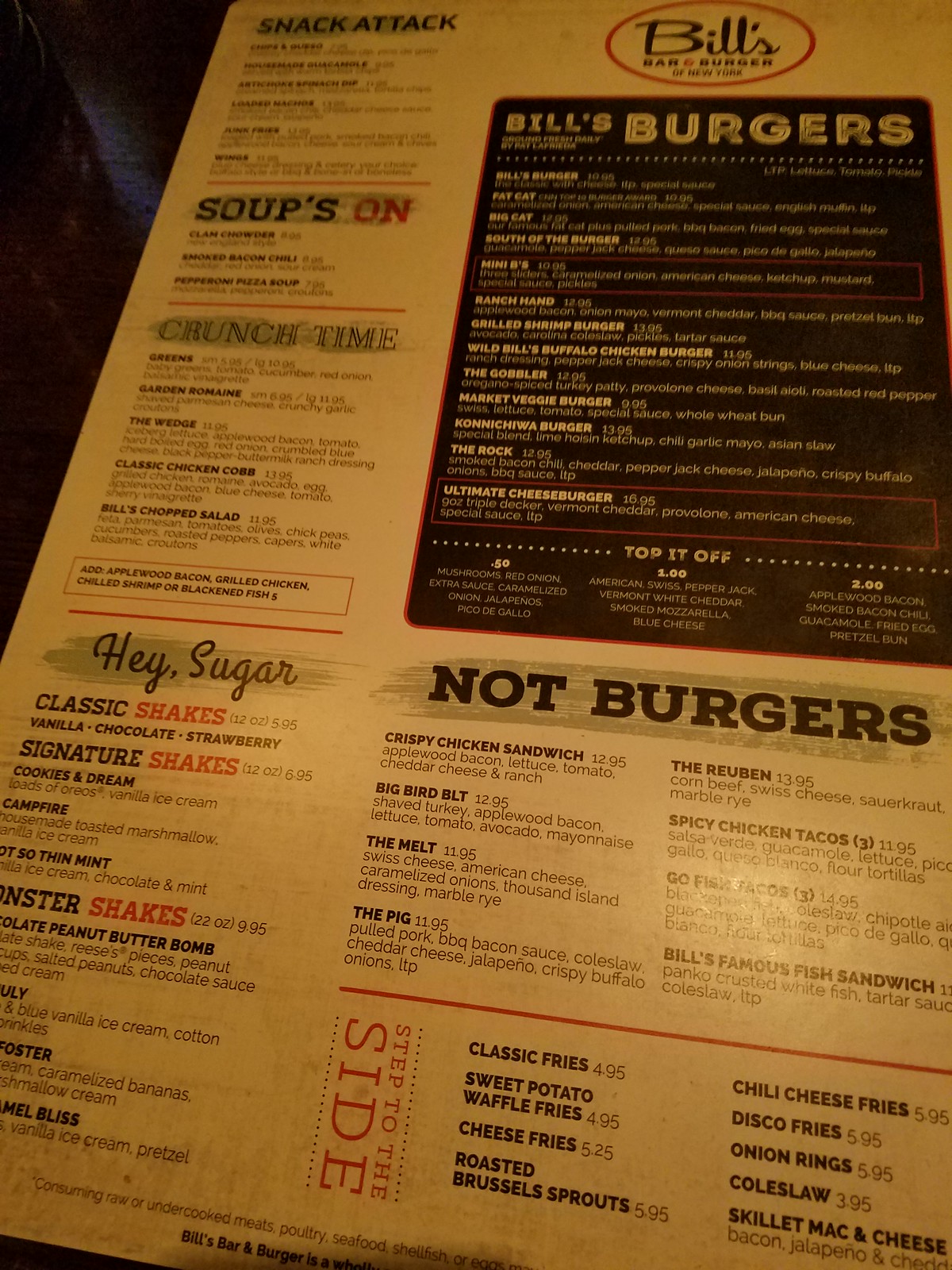This image captures a photograph of a restaurant menu from Bill's Bar and Burger, taken in an indoor setting. The menu, which has a notable rectangular, vertical layout, features a medium yellow-brown background with text in shades of red, burgundy, black, and brown. It is organized into several distinct sections: "Snack Attack," "Soups On," "Crunch Time," "Hay Sugar," "Bill's Burgers," and "Not Burgers." The menu appears relatively large and tall, suggesting a wide variety of options available to diners. The carefully chosen color scheme and structured sections contribute to a visually appealing and easy-to-navigate menu design.